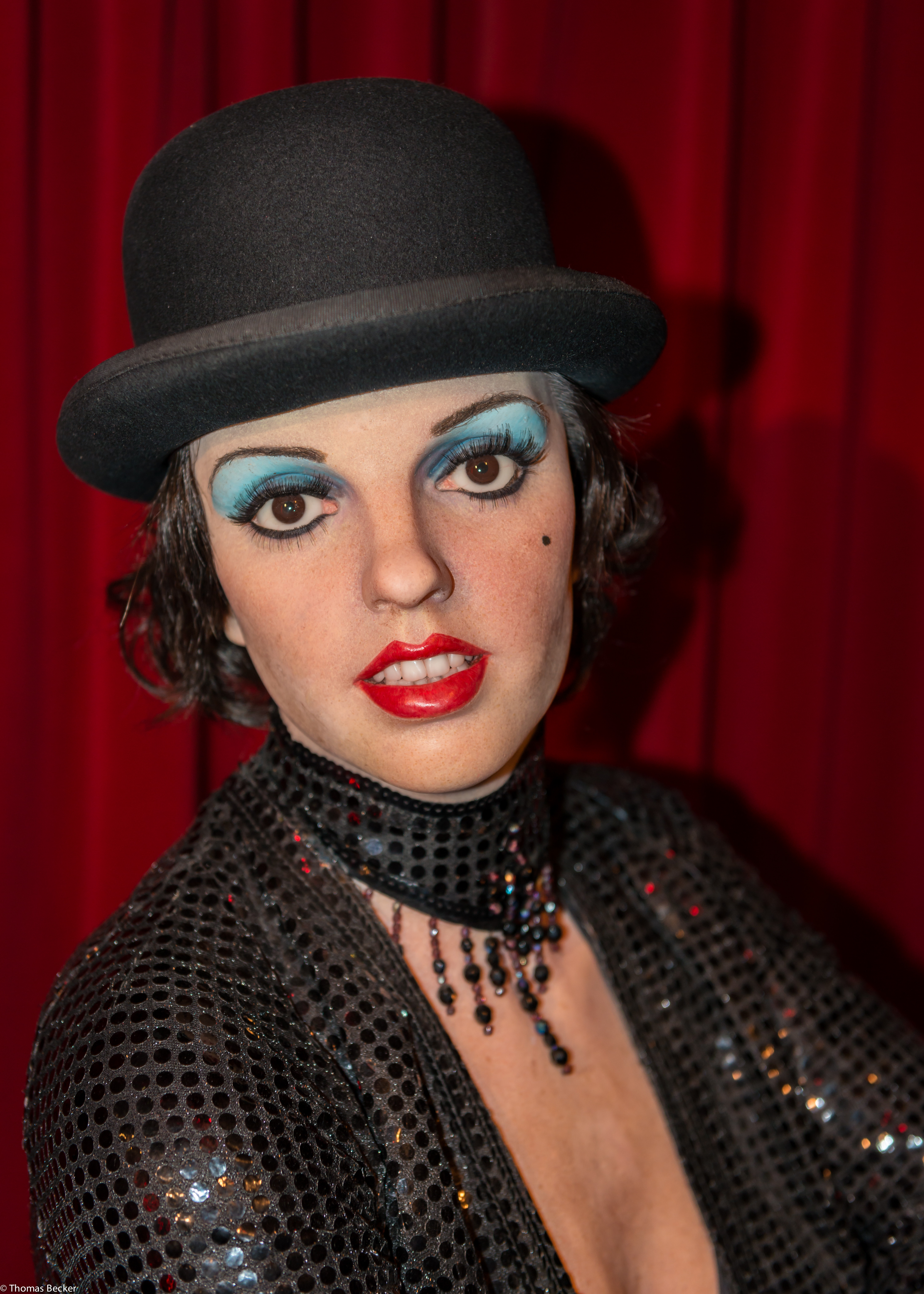This photograph captures a young Liza Minnelli prominently positioned at the center of the image. She exudes a striking presence with her dramatic makeup, which includes bright teal blue eyeshadow reaching up to her well-defined black eyebrows, and cherry red lipstick that highlights her slightly open mouth, revealing her teeth. A distinct beauty mark adorns her left cheek. Liza is wearing a black sequined bowler hat that complements her short black hair, which falls just past her ears. Her outfit is equally dazzling; she is dressed in a low-cut, black sequined V-neck blouse with a matching collar-necklace adorned with black jewels. The backdrop is a luxurious, heavy red curtain that adds depth and contrast to the scene, along with a shadow cast by Liza, visible in the center-right of the image.